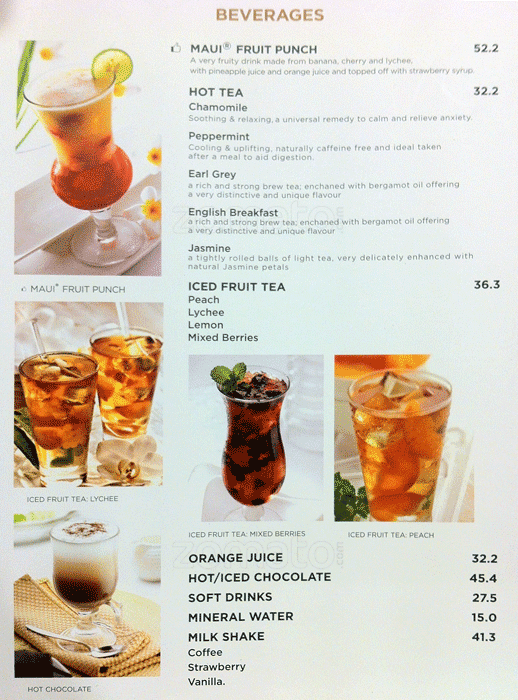The color photograph captures a page from a drink menu, predominantly white with a light gray background and brown text that reads "Beverages" at the top right. This page, dedicated to beverages, lists several drink options with prices. At the top, the Maui Fruit Punch is priced at 52.2 and is presented in a fancy margarita-style glass with a lime on the rim, adorned with small flowers and a green leaf. The menu also lists Hot Tea (32.2) in varieties such as chamomile, peppermint, earl grey, English breakfast, and jasmine. Further down, Iced Fruit Tea is available for 36.3 in flavors including peach, lychee, lemon, or mixed berries. Other options include Orange Juice (32.2), Hot or Iced Chocolate (45.4), Soft Drinks (27.5), Mineral Water (15), and Milkshakes (41.3) with choices of coffee, strawberry, or vanilla.

The menu features five photographs of drinks on the left side. These include the Maui Fruit Punch at the top, followed by images of Iced Fruit Tea Lychee and Iced Fruit Tea Mixed Berry. A photograph of Hot Chocolate shows a drink topped with whipped cream and chocolate. An additional photo features Iced Fruit Tea Peach, indicated by the presence of earth-toned hues in the images. The drinks vary in presentation, contributing to an elegant and inviting visual appeal on this sophisticated beverage menu page.